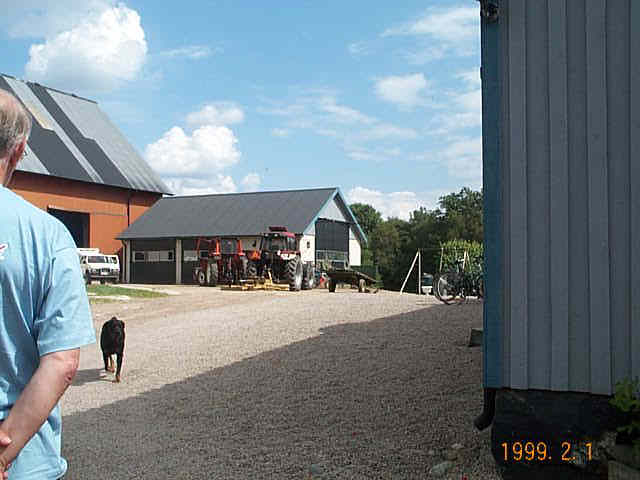In this 1999 photograph taken outdoors, we see a scene of what appears to be a farm on a sunny day with a blue sky dotted by white clouds. Dominating the image is a large, red-orange barn with a sloped gray and black roof. Adjacent to the barn is a white truck, seemingly with its trunk open, and various pieces of farm equipment, including red tractors with large wheels. There’s also an open farm building that looks like a garage, nestled next to the barn. 

In the foreground, on the left, stands an older man with gray hair, a bald spot, and glasses, clad in a blue short-sleeved shirt. Only the upper half of his body is visible as he faces away from the camera with his hands behind his back. Walking on a gravel path towards the man is a black dog, possibly a Labrador. Additional details in the background include trees with green leaves and, on the right side, a glimpse of another building with a black roof. The remnants of a few bicycles are also set up around the area, underlining the rural setting of the scene. The bottom right corner of the photo is marked with the date "1999-2-1," overlapping the image itself.